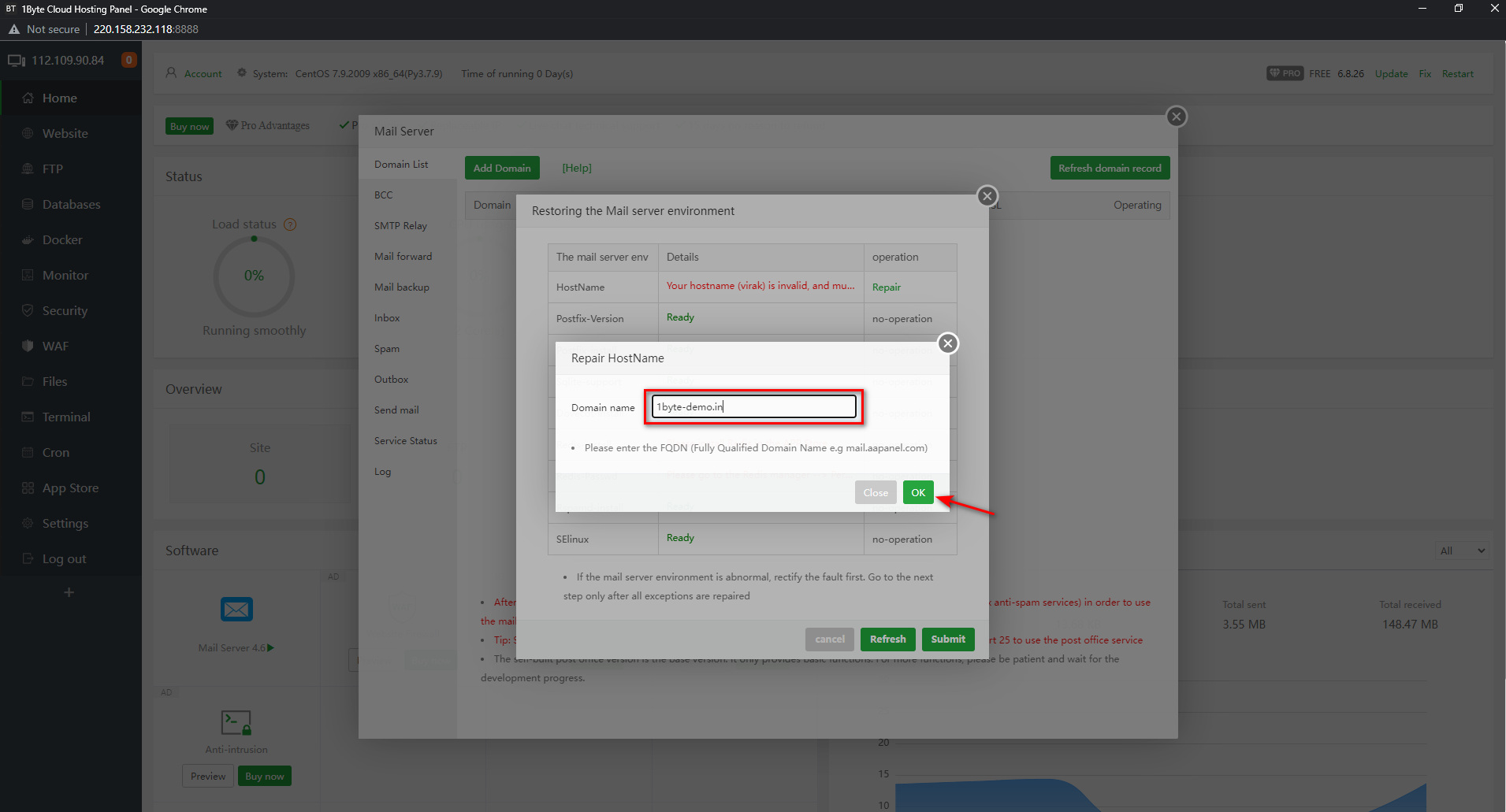The image displays a detailed and layered view of multiple web pages open in Google Chrome. At the bottom layer is a Cloud Hosting Panel displaying an account page, covered by a mail server page. Above it is a page for restoring the mail server environment, and at the top is a white page focused on repairing the host name. 

Each lower layer has a gray haze, making them difficult to read. 

On the topmost white page, there is a header strip in gray with the text "Repair Host Name" on the left side and a circle with an X on the right side, indicating a close option. Below the header, a data field labeled "Domain Name" contains the text "BYTE-DEMO.IN," outlined in black and encased in a red outline added by a photo editor. 

Beneath this field, an instructional message reads, "Please enter the FQDN (fully qualified domain name), e.g., mail.aapanel.com." 

At the bottom right corner of this page are two buttons: a green "OK" button with white text and a close button. A red arrow points to the "OK" button, suggesting the image is being used for educational purposes.